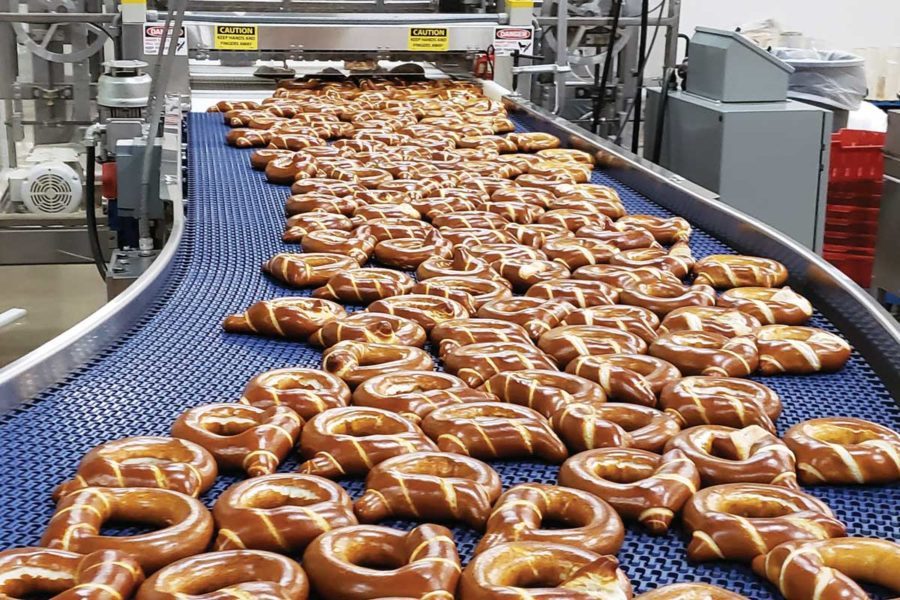The image showcases a photorealistic scene of a blue rubber conveyor belt in an industrial factory setting, transporting a large quantity of glossy, unsalted, and well-baked pretzels toward a background machine. The pretzels are uniformly tied and shaped with a knot at the bottom, and their dark brown appearance suggests they are almost ready for packaging. Flanking the navy blue conveyor belt, which has ventilation holes, are stainless steel sides, adding to the industrial look. Red crates and a fan can be seen to the right and left of the belt respectively, along with various gray machinery and caution signs advising safety. In the background, there's a garbage can and other operational panels, though no workers are present in the frame. The scene captures a moment in the pretzel production line before the salting process.